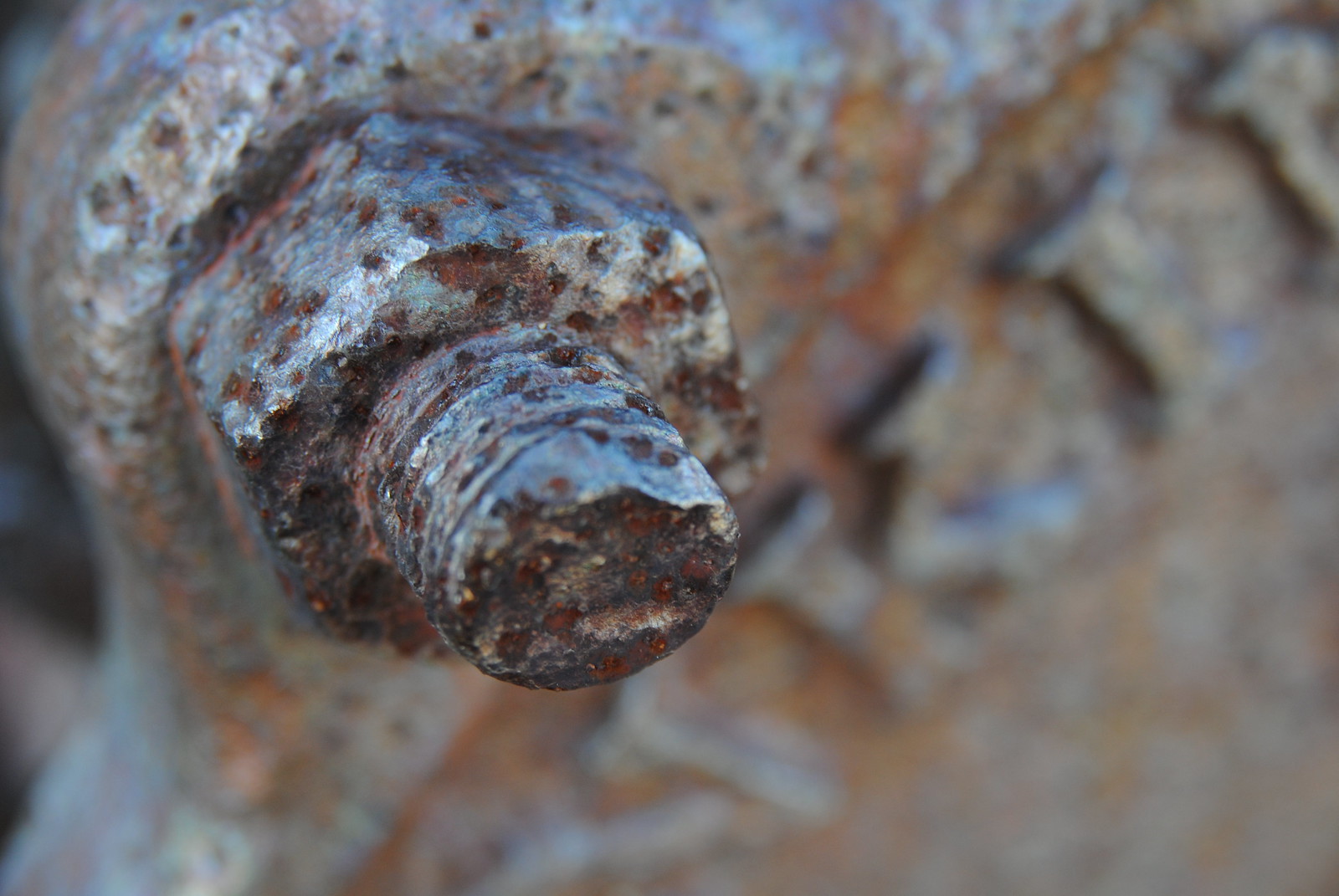This photograph is a close-up, macro shot of a weathered and heavily rusted nut and bolt. The nut is screwed onto the bolt, both of which display significant chipping and rust, giving them a reddish-brown appearance. The two components are attached to a larger, silver-colored metal object that is also speckled with rust, indicating prolonged exposure to the elements. Engraved at the bottom of this metal, the letters "K" and "I" are discernible, though the surrounding area is blurred, obscuring the full text. The photograph is sharpest around the nut and bolt, with the sides becoming progressively blurrier, focusing attention on the central, rusted hardware. In the background, hints of another metal structure are visible but indistinct, adding to the aged and outdoor-worn character of the scene.